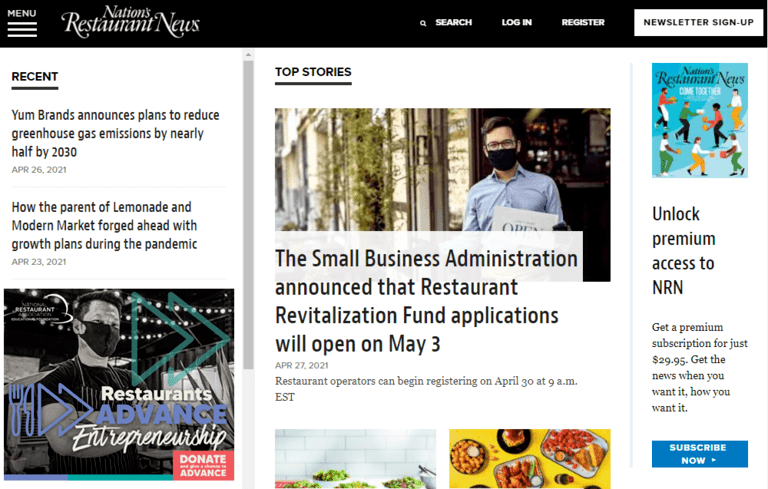This screenshot captures the homepage of a website. At the very top, there is a sleek black banner with white text. On the upper left side of this banner, the word "Menu" is displayed, accompanied by three horizontal white bars, indicating a clickable menu. Next to this, in white font, is the title "Nations Restaurant News." Moving further to the right, a magnifying glass icon followed by the words "Search," "Login," and "Register" are also in white text. Central to this top section, there is a prominent white rectangle featuring the phrase "Newsletter Sign Up" in black font.

Beneath this banner, the main webpage unfolds against a white background. On the left side, there is a scrollable menu. This menu starts with the word "Recent" in bold black font. It is followed by several headlines and accompanying dates. The first headline reads, "Yum Brands announces plans to reduce greenhouse gas emissions by nearly half by 2030," with a timestamp in gray font indicating "April 26, 2021." Another headline positioned below states, "How the parent of Lemonade and Modern Market forged ahead with growth plans during the pandemic," dated "April 23, 2021" in gray font. At the bottom of this section, there is an advertisement banner that reads "Restaurants Advanced Entrepreneurship."

This detailed description highlights the key elements and layout of the webpage, providing a comprehensive visual understanding of the screenshot.